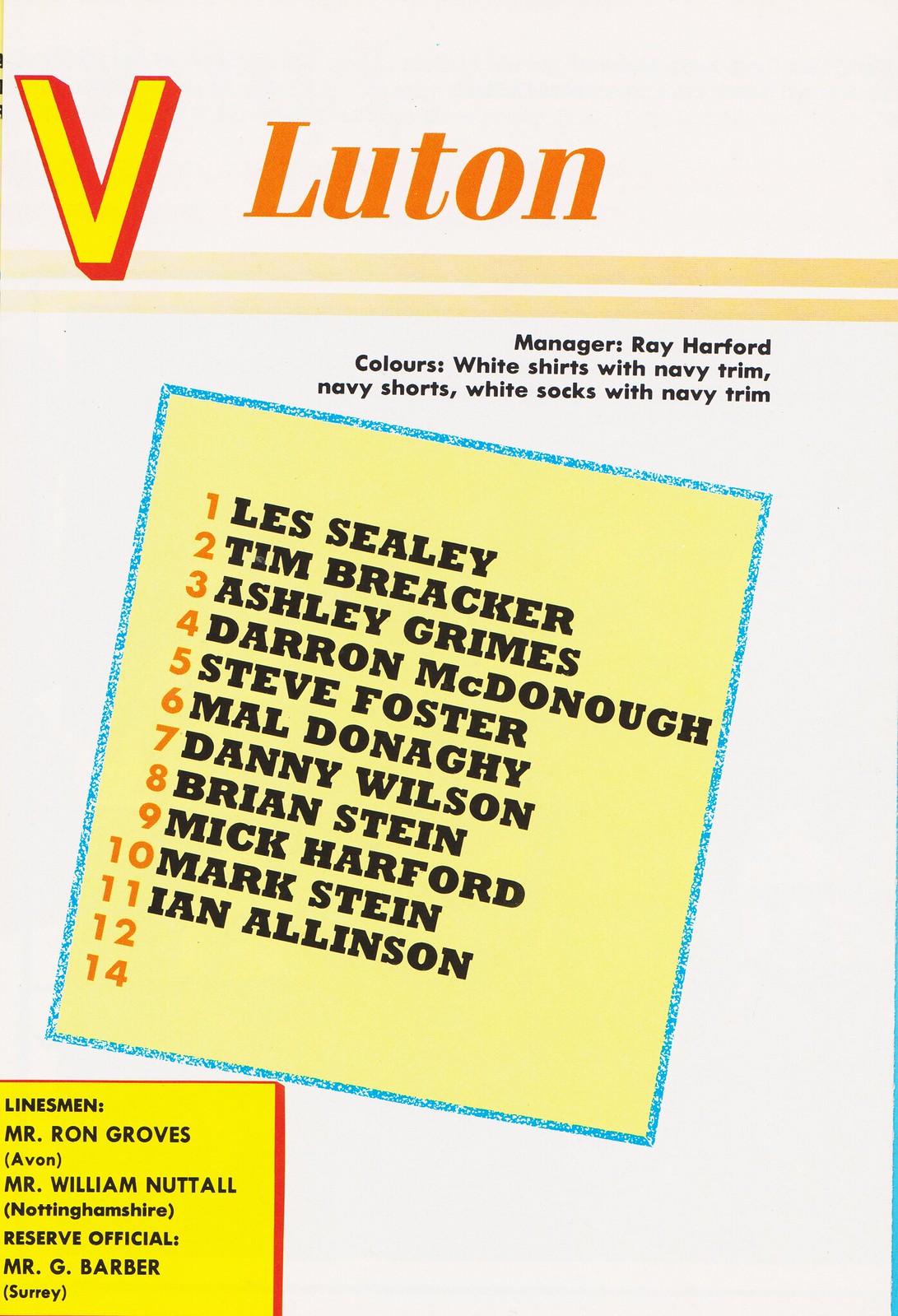This image features a cut-off section of a team roster, presumably from a soccer magazine or program for the team Luton. The background is an off-white color. Dominating the top left of the page is a large yellow "V" with a red shadow, partially cut off. To the right of the "V," in orange text, it reads "LUTON." Below this are two light yellow stripes, with text beneath them stating "Manager Ray Harford" and describing the team colors: white shirts with navy trim, navy shorts, and white socks with navy trim.

In the center of the image is a yellow box, slightly tilted to the right, with a light blue border. This box lists the player roster in bold black text with orange numbers: 1. Les Seeley, 2. Tim Breaker, 3. Ashley Grimes, 4. Darren McDonough, 5. Steve Foster, 6. Mal Donahue, 7. Danny Wilson, 8. Brian Stein, 9. Mick Hartford, 10. Mark Stein, and 11. Ian Allison. There are also spots for a 12th and a 14th player, though no names are listed next to those numbers; notably, the 13th spot is missing, perhaps due to superstition.

At the bottom of the image is another yellow box with a red outline containing the names of the linesmen and reserve official in small black text: "Linesman, Mr. Ron Groves, Avon," "Mr. William Nuttall, Nottinghamshire," and "Reserve Official, Mr. G. Barber, Surrey."